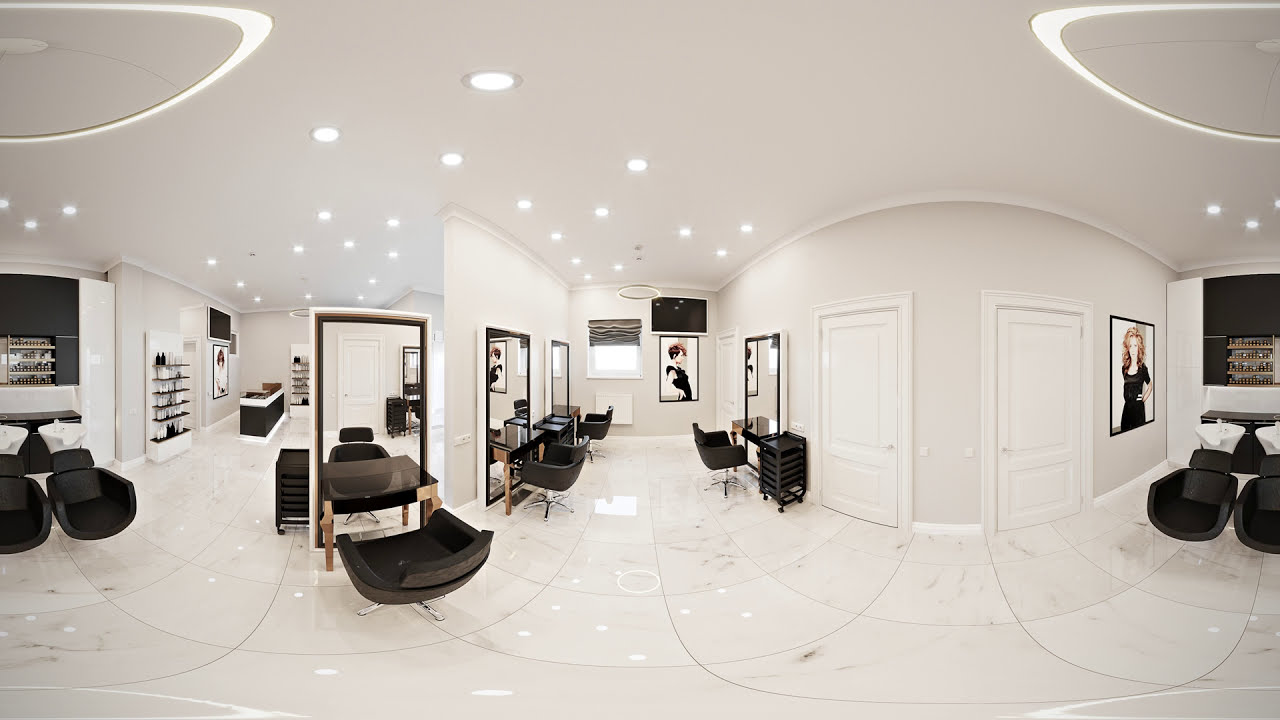This photograph captures the modern and elegant interior of a bright, well-lit beauty salon. The space features glossy white marble floors with gray streaks and is sectioned into three different rooms by white walls and white doors. Each room is illuminated by recessed lighting and circular ceiling decorations, creating a cheerful and sophisticated ambiance.

The center room houses several styling stations, each equipped with a floor-length mirror, a dark-topped table with brown legs, and a black chair on wheels placed in front. Scattered single lights add to the brightness. In total, there are nine chairs visible throughout the salon. The left room includes a front desk in black and white, with additional seating areas.

Framed black-and-white photographs of women with elaborate hairstyles adorn the walls, adding a touch of artistic flair. Shelves stocked with shampoos, mixers, and beauty products are strategically placed around the rooms, ensuring everything needed is within easy reach. The overall décor is sleek and modern, evoking a sense of professional luxury.